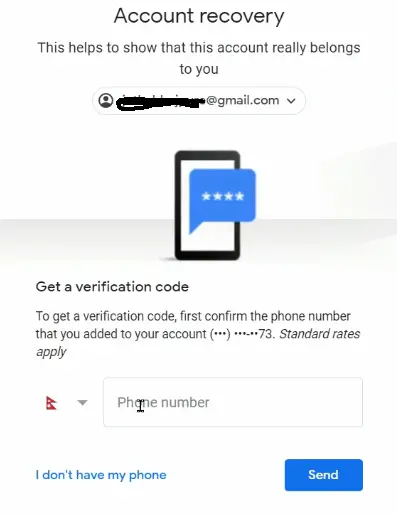The image displays an account recovery interface set against a white background. Central to the image is a profile icon next to a partially obscured name and a beginning of an email address ending with "@gmail.com," indicating that this is a recovery procedure for a Google account. Below the email address is a notification prompting the user to get a verification code by confirming the phone number associated with the account. The obscured phone number is presented as (*******-**73).

In the lower part of the interface, there is a text box labeled "Phone Number," which contains a blinking black cursor, ready for user input. Below the text box is an option in blue text that reads, "I don't have my phone."

On the right side of the text box, there is a blue button with the word "Send" written in white. Surrounding elements include a blue comment icon with four white stars and standard message rates warning in italics. Additionally, there are two red downward-facing triangle icons, one partially gray, presumably signifying errors or alerts.

The interface emphasizes user verification through the entered phone number as a means of account recovery, highlighting the steps required for the user to regain access to their account.